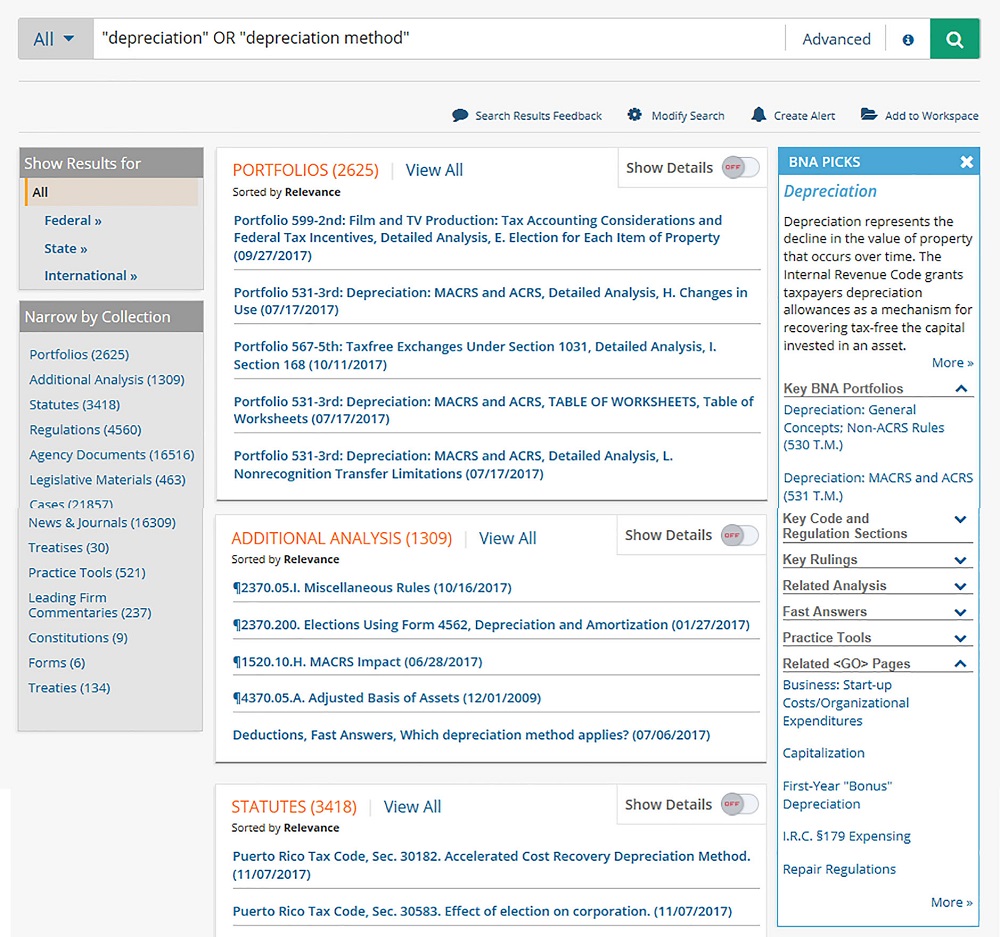The image depicts a comprehensive law research website, resembling platforms such as BNA, Lexis, or Nexis. At the top of the interface, there's a prominent search box where a user has entered the search terms "depreciation" and "depreciation method," both enclosed in quotation marks to ensure precise search results. Adjacent to the search box is a search icon symbolized by a magnifying glass, along with an advanced search bar offering various refinements commonly found on legal research websites.

Beneath the search area, there's a series of drop-down menus that facilitate user interaction with the search results. These options include providing feedback on the search results, modifying the search parameters, creating alerts for newly added cases related to the search terms, and adding the current search to the user’s workspace for future reference.

The search results are displayed in a tri-column format, detailing federal, state, and international results. This layout allows users to specify the jurisdictional scope of their research. Additionally, the interface offers a feature called "collections," which organizes related documents and information, helping users to narrow down their focus based on specific groupings of the search terms. The meticulous design ensures that legal professionals can efficiently conduct comprehensive research on topics such as depreciation and depreciation methods.